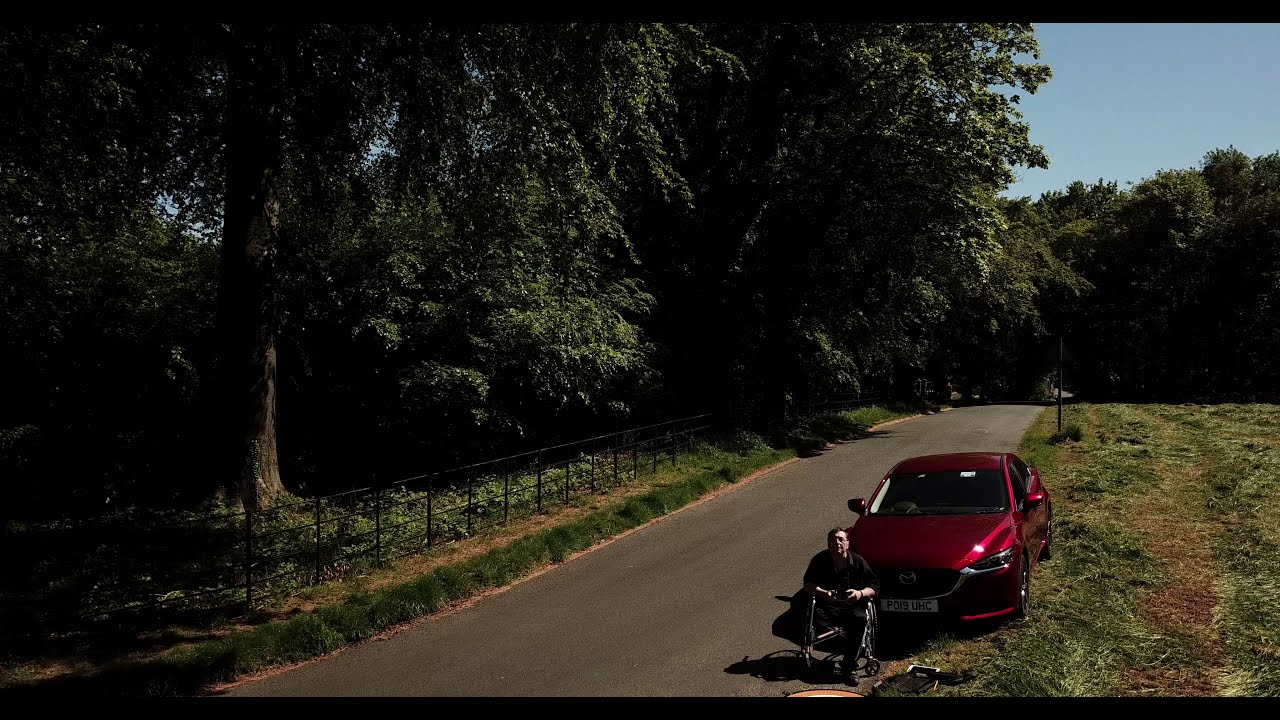In this detailed photograph set on a country road during daytime, the scene is dominated by a clear blue sky and a rugged rural landscape. The road, which uniquely appears green in color, runs through the center of the image. To the right side of the road, a shiny dark red car is parked with a white license plate showing black letters. In front of this car, an older man is seated in a wheelchair, wearing a dark short-sleeved shirt, and he looks directly at the camera. The camera is positioned at a distance from him, capturing the full scene.

On the far right side adjacent to the road, there is a ground covered with a mix of green and brown grass. On the left side of the road, a black metallic fence runs parallel, stretching from the bottom left and proceeding towards the center right of the photograph. Beyond this fence stands a large, dominant tree with a sturdy trunk and cascading branches that nearly reach the top of the image, along with an array of other trees and abundant leaves filling the background. The entire image is horizontally oriented, showcasing a tranquil, natural setting indicative of a country road.